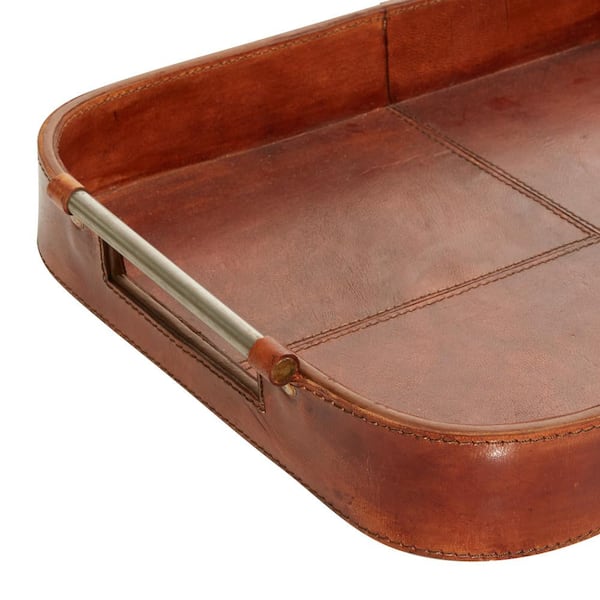The image features a close-up shot of a faux leather serving tray, partially visible and positioned against a stark white background, likely under studio lighting. The tray is a deep caramel color with a slightly worn appearance, highlighting detailed brown machine stitching along the edges and interior sections. The visible portion of the tray emerges from the right side of the photo and is flipped upside down, revealing its underside. The rectangular tray has curved corners and a sturdy metal handle on the side, which is cylindrical and silver with a small rectangular opening for finger grip. This handle allows for easy lifting. The tray's interior is divided into rectangular sections by triple stitch lines, enhancing its intricate design.